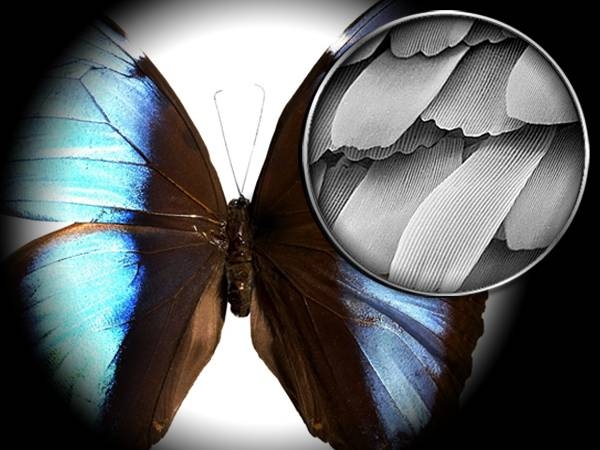This image features a stunning butterfly with intricate wing details and vibrant colors. The butterfly's body is brown, and its black antennae are prominently visible in the center. The wings, starting near the body, are dark brown or black and transition into a darker blue band that extends into a striking fluorescent turquoise and bright blue towards the outer edges. The wings have a lacy appearance accentuated by a black halo-like border that gives the impression of being viewed under a microscope.

On the right side of the image, there's a magnified inset detail that dramatically zooms into the wing structure. This black-and-white close-up reveals the intricate scales of the wing, showing them as overlapping, almost shingle-like formations with thin, vertical lines running through each scale, emphasizing their texture and layered pattern. These fine details highlight the complex and delicate architecture of the butterfly's wings, making the entire image spectacular and captivating. The background is gray, complementing the butterfly's vivid colors and further enhancing the overall visual impact.